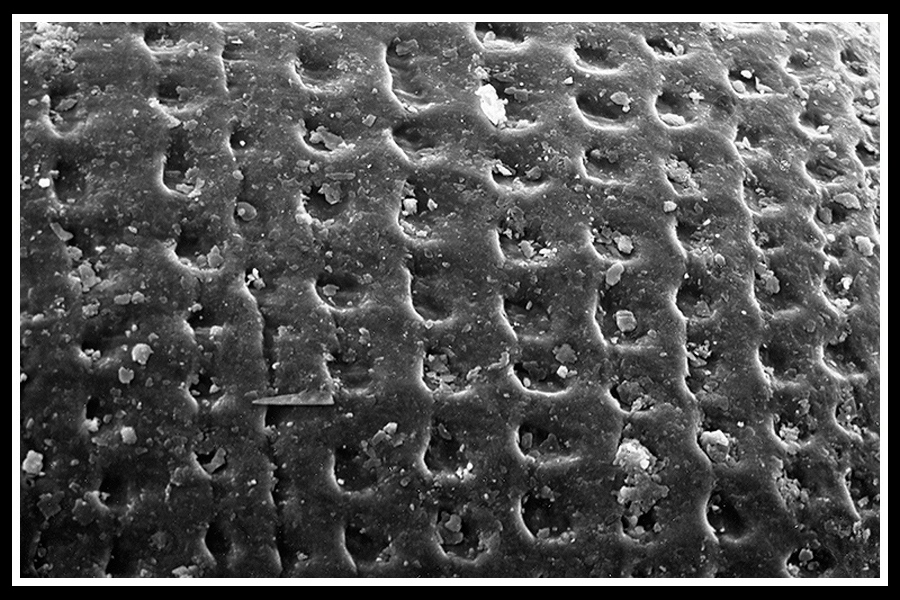This is a horizontally aligned black and white photograph with a distinctive white and black double border framing it. The image is somewhat ambiguous but appears to depict a textured surface resembling a piece of material with numerous small, circular indentations arranged in rows. These indentations might be likened to footprints or pockets. Scattered throughout the image are small, rock-like chunks, adding to the textured appearance. The overall coloration is shades of gray, giving it a slightly grainy, almost real and somewhat computerized feel. The subject in the photo could be under a microscope or some close-up view, but the exact nature is unclear. There's a notable comparison to a piece of food such as peanut brittle or a cookie, which might be where the textural imprints and sprinkling effect come from. The photo lacks any date, location, or time information, and there are no people visible in the image.